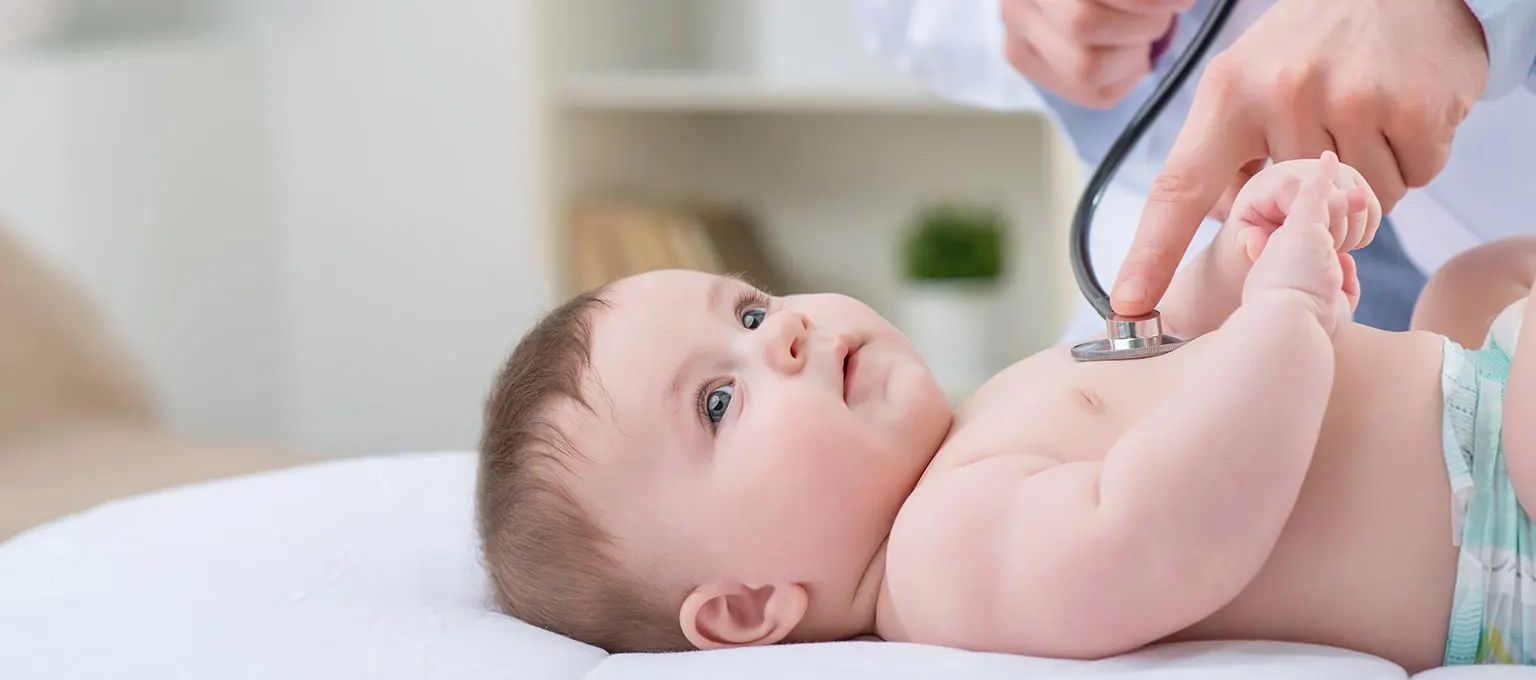The photograph captures a detailed scene of a medical examination of a baby boy with fair skin. He is lying on his back on a white bed, wearing a light blue diaper. The baby, who has short brown hair and chunky, glossy-eyed arms, gazes upwards with a slightly dazed yet alert expression. His head is positioned towards the left, and his diaper is visible to the right. The focus of the image is on the doctor’s hands, which are lightly pressing a stethoscope against the baby’s chest, monitoring his heartbeat. The doctor, invisible apart from his hands and white lab coat, signifies a clinical setting. In the blurred background, there appears to be a shelf with a white cup containing green plants, along with a white cupboard and a beige chair, indicating the examination room's surroundings.